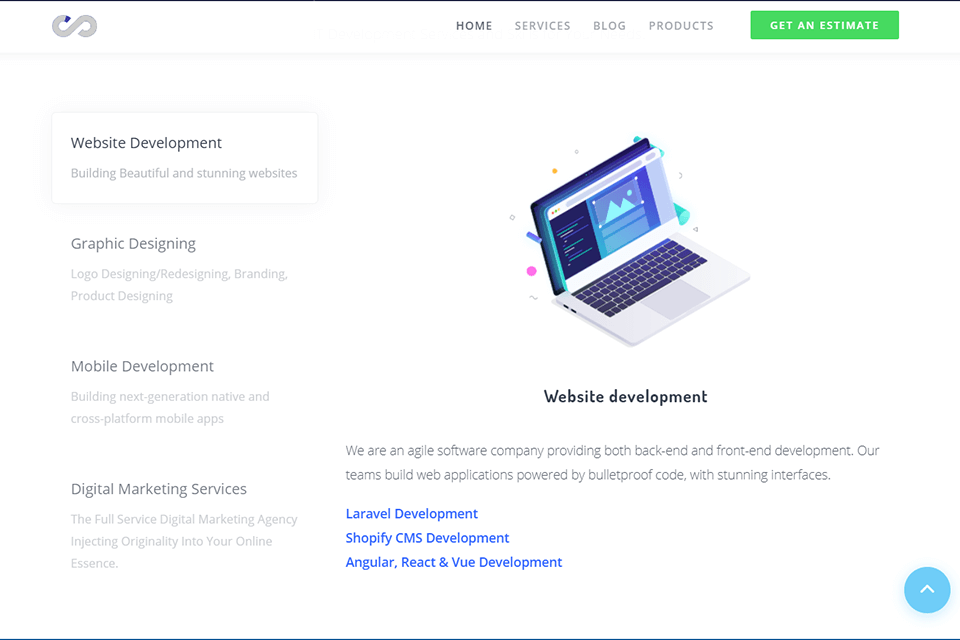On a pristine white background, the website’s navigation is displayed prominently at the top with sections labeled: Home, Services (in black and gray), Blog, and Products. Anchored on the right is a vibrant green rectangle bearing the text "Get an Estimate" in white letters.

Below this menu, a central image features a laptop screen displaying the phrase "Website Development." The accompanying caption declares, "We are an agile software company providing both back-end and front-end development. Our teams build web applications powered by bulletproof code with stunning interfaces."

To the right of the laptop image, in distinct blue text, various services offered by the company are listed: Laravel Development, Shopify Development, CMS Development (written in all caps), Angular Development, React Development, and Vue Development.

On the left side, another list details the company's wide range of expertise:
- Website Development: Building beautiful and stunning websites
- Graphic Designing
- Logo Designing/Redesigning
- Branding
- Product Designing
- Mobile Development: Building next-generation native and cross-platform mobile apps